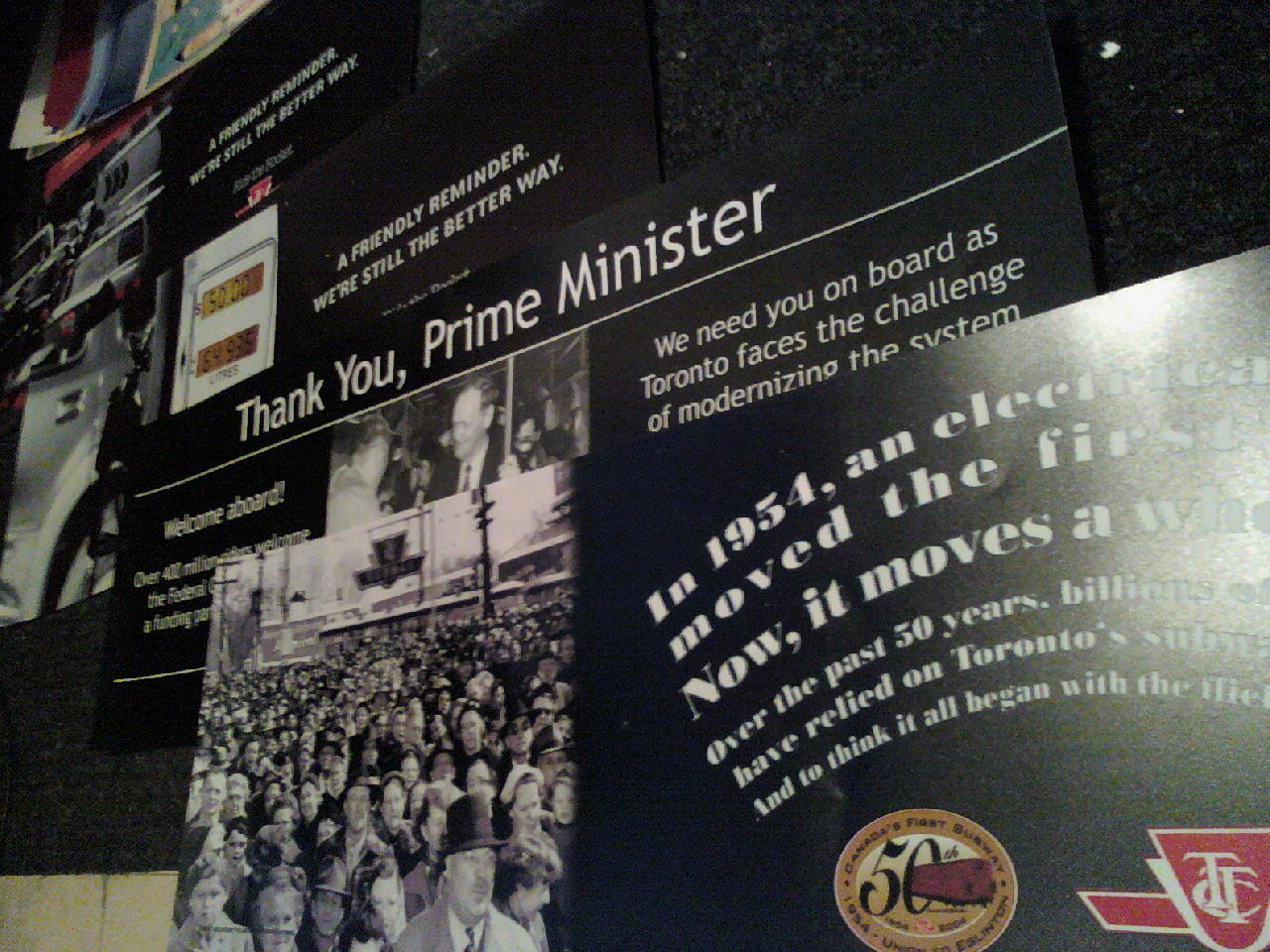The image captures a mural inside a museum or building, filled with various plaques and posters chronicling historical events, predominantly in black. The mural, in landscape orientation, features a montage of textual and photographic elements. Dominating the visual scene is a series of black-background panels adorned with stark white text. On the left, bold white lettering states "Thank You, Prime Minister," set against a dark background with an underlying black and white photograph of a crowd, presumably from a significant event. Central to the mural is a prominent section referring to the year 1954, adjacent to a black and white photograph depicting a crowd participating in what appears to be a political rally. Above this, in a white arc-shaped font, the partially visible text reads, "In 1954, an electrician moved the first blank and now it moves blank," with more text cut off to the right. At the bottom right corner, two logos are displayed: a gold ellipse and a red triangle with white lettering. There are additional truncated texts and images scattered throughout, enhancing the mural's photographic representational realism style. Overall, the mural melds historical imagery with textual elements to create a detailed, visually engaging documentation of significant events.